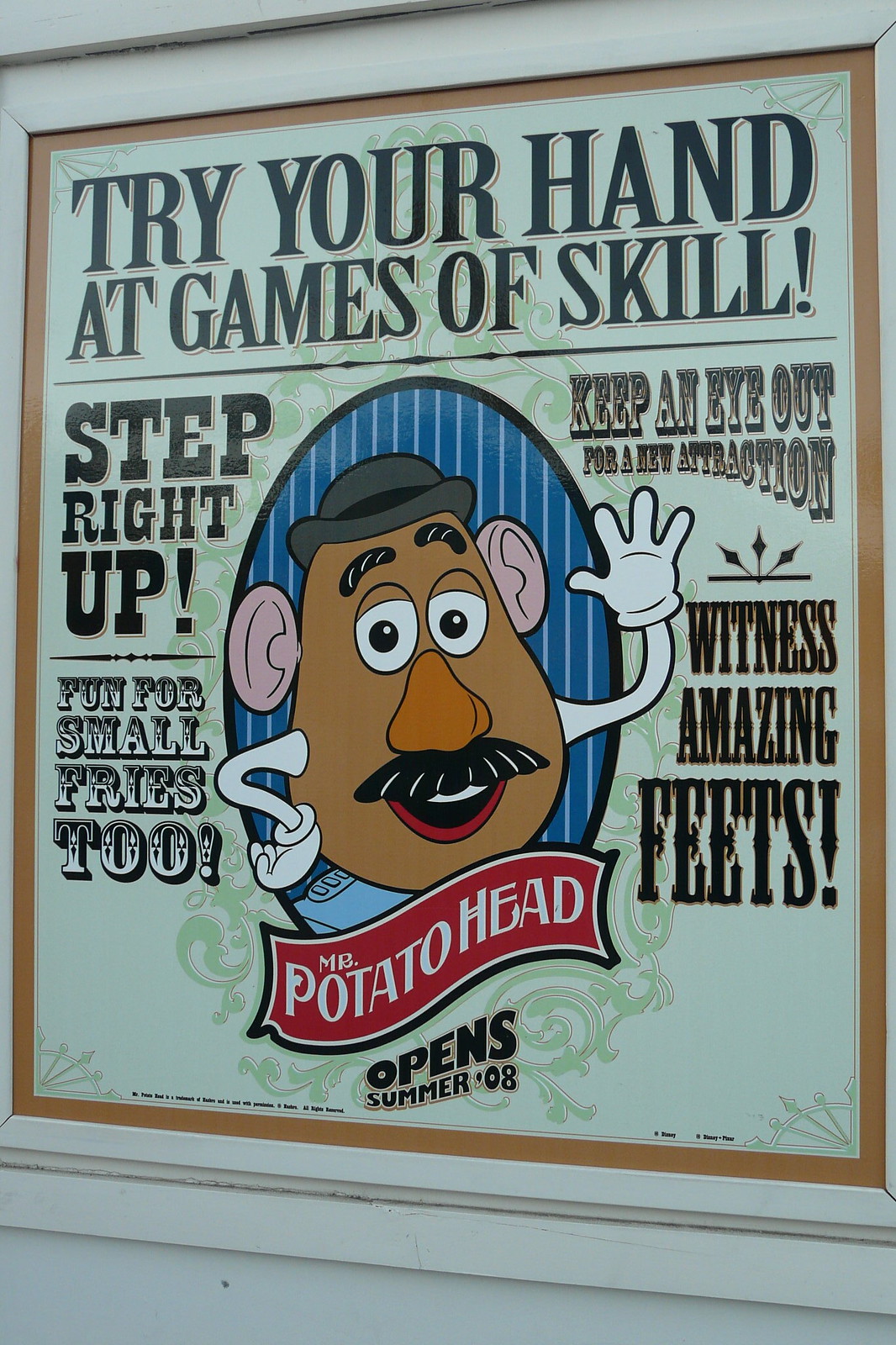The advertisement is a large, colorful sign plastered on the outside of a wall, promoting an upcoming attraction featuring Mr. Potato Head. Dominated by an old-timey theme, the ad captures attention with bold black text at the top that reads, "TRY YOUR HAND AT GAMES OF SKILL!" in all capital letters. In the center, a cartoonish Mr. Potato Head waves cheerfully, wearing a hat, a mustache, and sporting white gloves with big pink ears. Below him, a red banner prominently displays his name, "Mr. Potato Head." On the left side of the image, the text reads, "STEP RIGHT UP!" while on the right, it invites visitors to "KEEP AN EYE OUT FOR A NEW ATTRACTION." Further enhancing the carnival-like atmosphere, the bottom left corner announces, "FUN FOR SMALL FRIES TOO!" and the bottom right promises, "WITNESS AMAZING FEATS!" The advertisement closes with a note at the bottom announcing the opening date, "SUMMER 08."